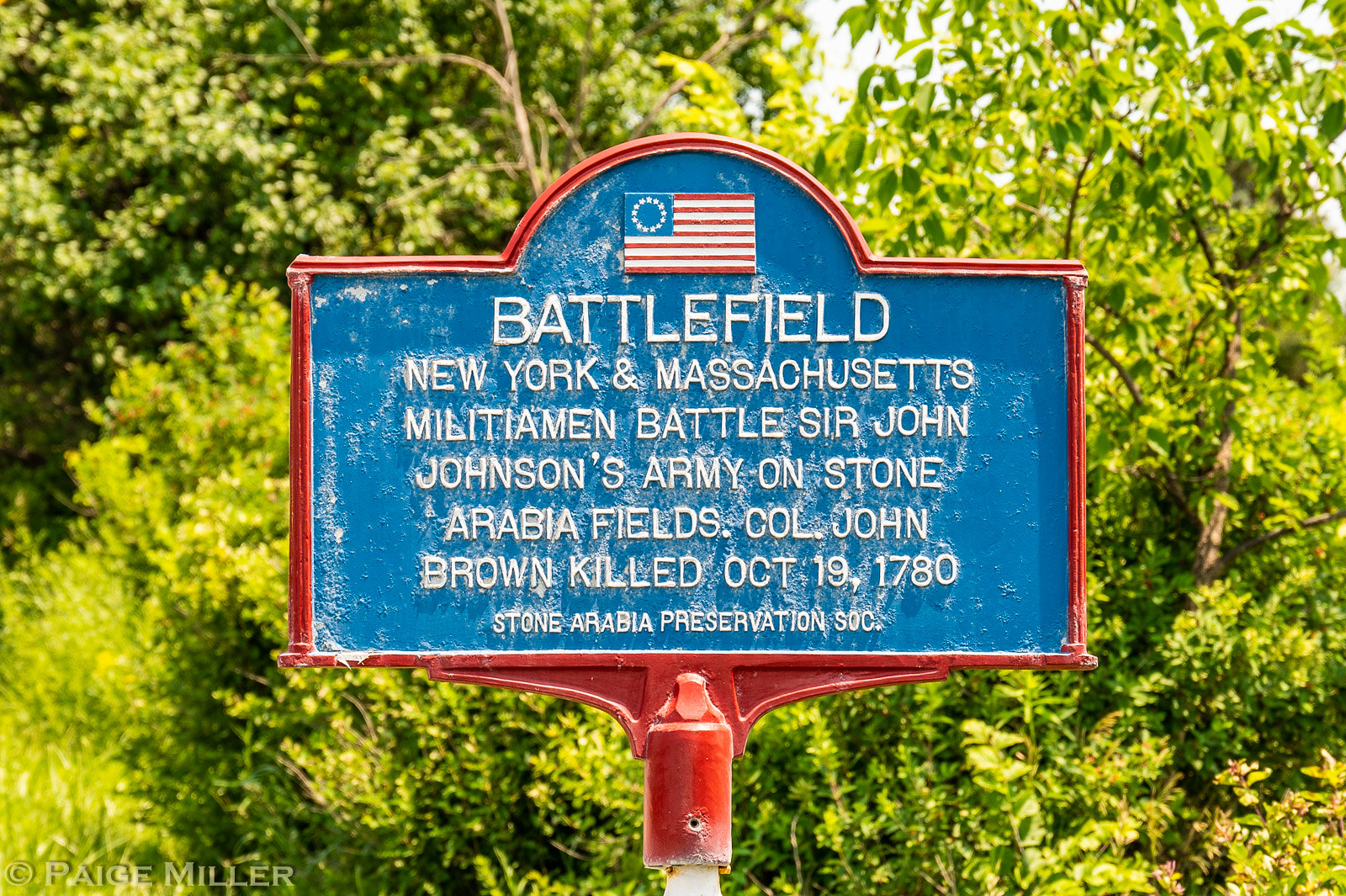The photograph captures a vivid outdoor scene with a strong emphasis on a historical memorial sign. Set against a backdrop of lush trees bathed in sunlight, the sign stands prominently on a red metal post, framed by a striking red border. The middle section of the sign features an old American flag with a circular arrangement of stars, placed above a deep blue background with raised white lettering. The text reads: "Battlefield, New York and Massachusetts. Militiamen battle Sir John Johnson's army on Stone Arabia fields. Colonel John Brown killed October 19, 1780." Below this, the sign is credited to the "Stone Arabia Preservation Society." The bright, clear day highlights the details of the scene, with patches of blue sky visible through the trees, enhancing the overall crispness and historical significance of the image.